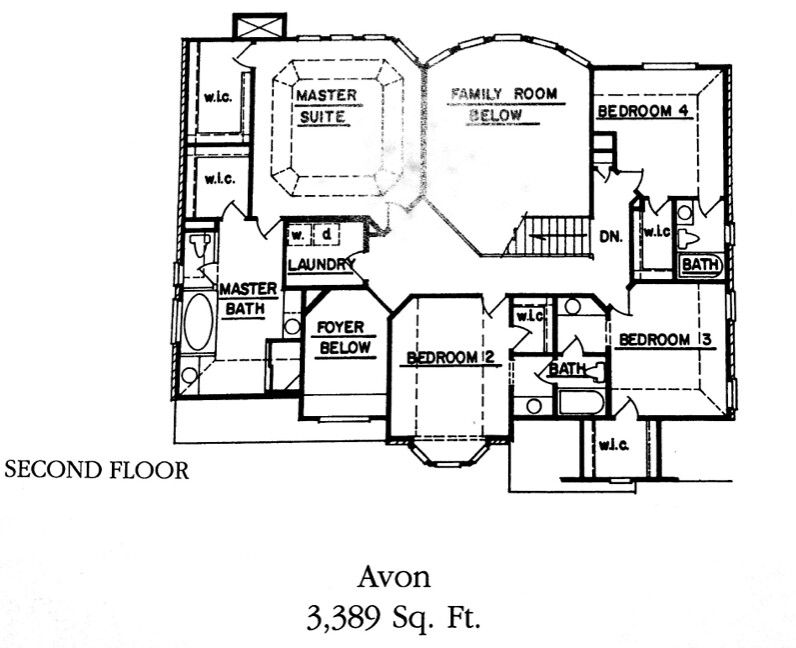Detailed Caption:

This detailed blueprint illustrates the second floor design of a 3,389 square foot residential dwelling named "Avon." The blueprint is predominantly rectangular, slightly wider than it is tall. Key elements of the second floor include:

- **Master Suite**: Located prominently with two spacious walk-in closets and an attached master bath.
- **Laundry Room**: Conveniently situated for easy access.
- **Bedrooms**: Bedroom number two, bedroom number three, and bedroom number four are strategically positioned.
- **Shared Bath**: A bathroom is placed between bedroom number two and bedroom number three.
- **Family Room Below**: Indicated on the blueprint between the master suite and bedroom number four, suggesting a double-height space that connects with the family room on the first floor.
- **Foyer Below**: Positioned below bedroom number two and next to the laundry room.

The layout emphasizes a well-thought-out flow for family living, balancing private and shared spaces efficiently.